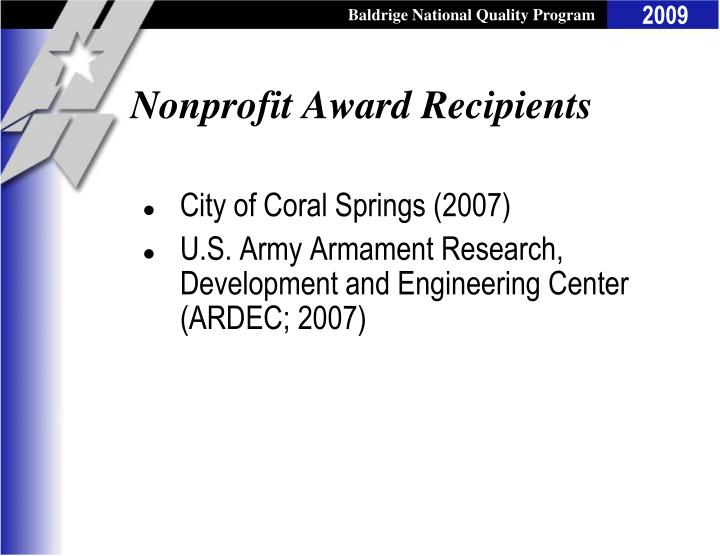This image appears to be a detailed graphic that resembles a PowerPoint slide or an ad. The background is white with prominent black text. At the top, there is a black banner reading "Baldrige National Quality Program" in white lettering. Adjacent to it, on the right, is a dark blue box containing the year "2009" in white letters. On the left side, there is a vertical blue border and a gray ribbon with a white star.

The main content in the body of the slide is titled "Nonprofit Award Recipients" in black cursive or print, followed by two bullet points. The first bullet point states: "City of Coral Springs (2007)." The second bullet point reads: "U.S. Army Armament Research, Development, and Engineering Center (ARDEC; 2007)." The overall design is highly structured, utilizing clear borders and distinct sections to organize the information.